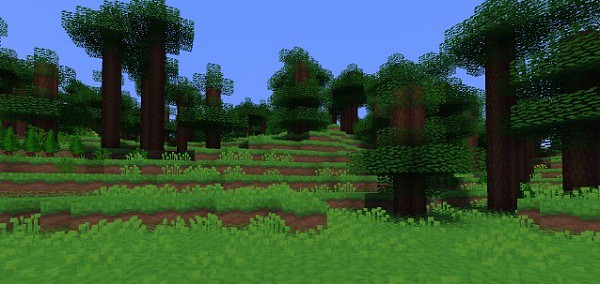This image depicts a vintage-style video game with a distinctive blocky design. The landscape is predominantly covered in vibrant green grass, interspersed with patches of scattered flowers, which also appear green. The terrain features several dirt patches, creating a mosaic of browns and greens that makes for a visually engaging ground layer. The trees within this virtual world are peculiar in appearance; each has a brown trunk and segmented, rounded canopies of lush green foliage. Some of the trees reach up to form tall canopies, adding vertical diversity to the environment. The overall aesthetic evokes a nostalgic, retro gaming atmosphere.